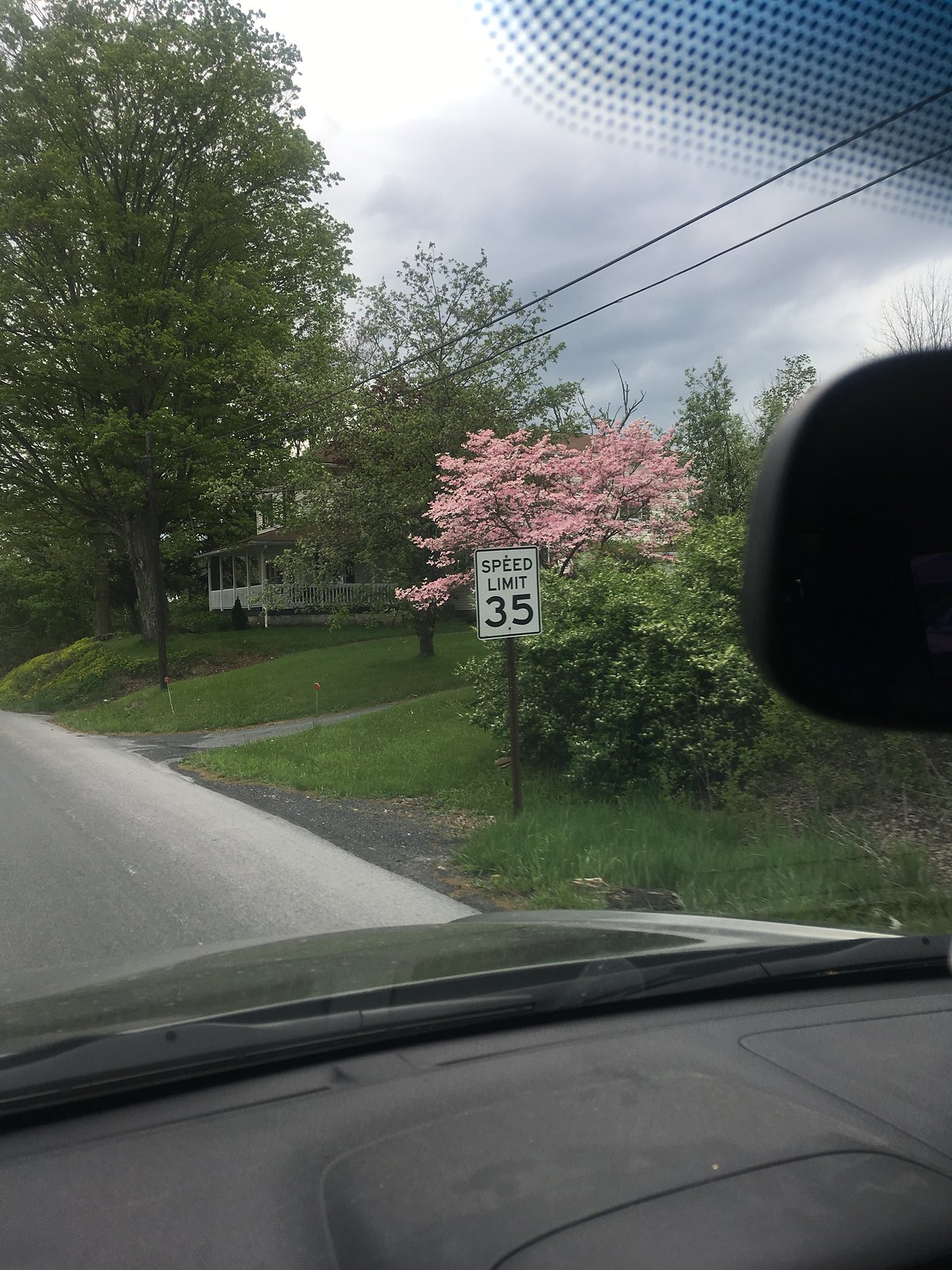This vertically oriented color photograph captures a serene spring scene from the interior of a car, taken through the windshield from the driver's seat. In the lower portion, the car's dashboard is visible, anchoring the viewer's perspective. Beyond the windshield unfolds a picturesque street lined with lush, green grass and several trees, including a striking pink flowering tree that adds a burst of color to the composition.

In the distance, a white house peeks through the foliage, evoking a sense of suburban tranquility. A speed limit sign displaying "35 mph" stands along the roadside, emphasizing the calm, residential nature of the area. The sky is slightly overcast, with light, pastel-colored clouds adding depth and softness to the scene. Telephone lines stretch diagonally across the sky, further enhancing the sense of everyday life.

To the left center of the image, the car's side-view mirror appears slightly blurred, hinting at the photographer’s position and adding an element of authenticity to the setting. The road itself curves to the left, inviting the viewer to imagine the journey ahead. The overall color palette is soft and calming, perfectly capturing the peaceful ambiance of a spring day.